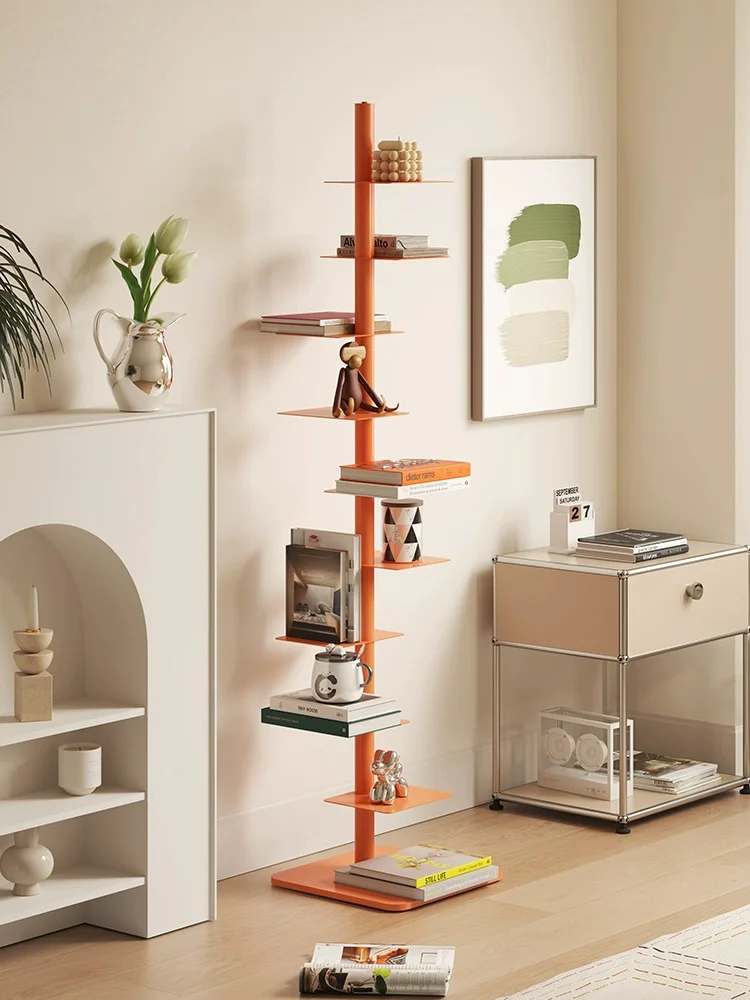The image depicts a meticulously arranged living room showcasing a standout, vertically-aligned, dark brown wooden shelf unit positioned against a light tan wall and atop a light brown wood-tiled floor. This central unit features a sturdy, square-shaped brown base from which a tall, brown pole extends vertically. Attached to this pole, staggered on alternating sides, are small, square brown shelves holding an assortment of items. These items vary from books and figurines on the lower shelves to a coffee mug and more books on the upper shelves, contributing to a visually appealing and organized setup.

To the left of this central shelf is a white shelving unit with an arch cut-out that houses several horizontal shelves, each bearing a variety of objects, including a silver water pitcher filled with tulips on the mantelpiece, enhancing the aesthetic appeal of the room. Meanwhile, on the right side of the main shelf, there is a small, cube-like light brown drawer with a knob handle. Adjacent to this drawer stands a small table laden with books and other decorative items, above which hangs a painting characterized by abstract splash patterns.

In the foreground, a cozy corner with a partial view of a rug and scattered magazines completes the homely atmosphere of the living room. Overall, the carefully curated elements and thoughtfully placed decorations create a harmonious and inviting living space.